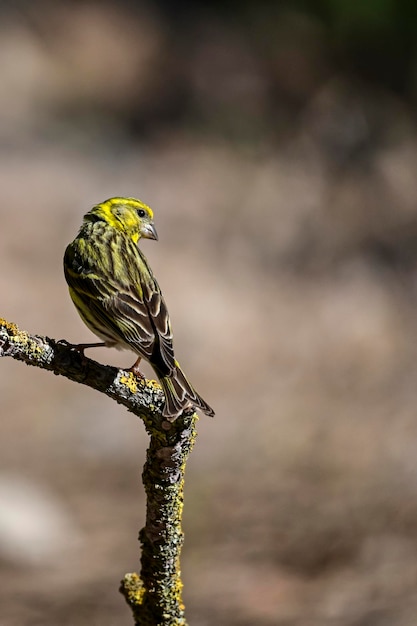The image features a small bird perched on a mossy, somewhat worn, and crusty tree branch situated on the left side of the photograph. The bird, striking in appearance, has a bright, brilliant yellow head with subtle gray markings. Its black eye and light-colored beak are distinctly visible as it turns its head slightly back toward the right, presenting a clear profile to the camera. The neck shares the same vivid yellow hue as the head, leading down to predominantly black wings accented with white and tiny bits of yellow. Its tail continues the pattern of black and white. The background is blurred, showcasing a mix of beige and black tones, which contrasts with and highlights the bird and branch in the foreground.